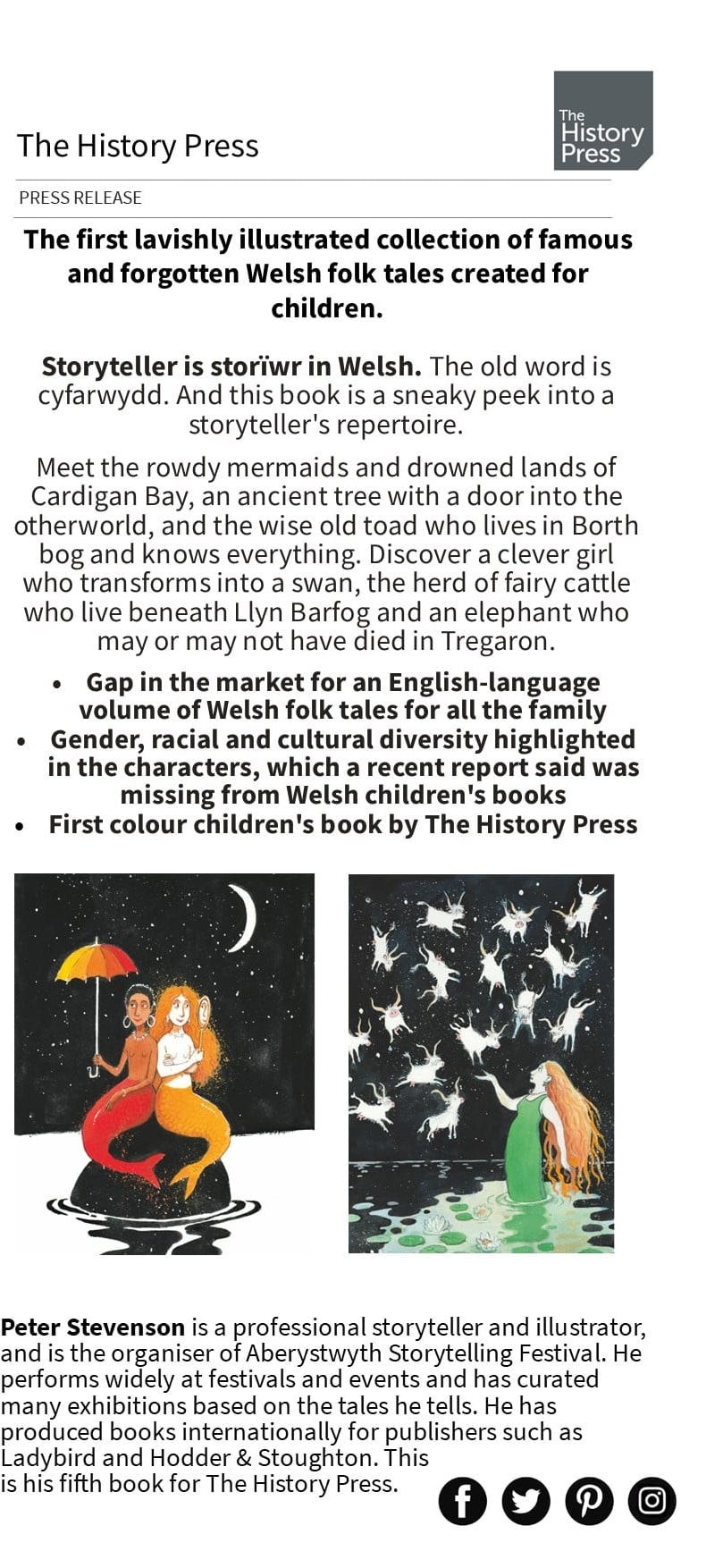This image is of a digital press release from The History Press, detailing their latest publication, "The First Lavishly Illustrated Collection of Famous and Forgotten Welsh Folktales Created for Children." The title is prominently displayed at the top, underlined by the tagline "Press Release." Below, we gain insight into the content of the book: an enchanting window into the world of Welsh folklore. This collection offers a colorful journey through tales of rowdy mermaids dwelling in the drowned lands of Cardigan Bay, an ancient tree with a doorway into the otherworld, and a wise old toad in Borthbog who knows everything. Additional stories include a clever girl who transforms into a swan, a herd of fairy cattle living beneath Llyn Barfog, and an elephant whose fate in Tregaron remains a mystery.

Illustrations accompany the text, adding visual appeal and context to these mythical tales. On the left, an image depicts two mermaids sitting on a rock at night, with one holding an umbrella. Another illustration shows a woman in a green dress standing in water, raising her hand to the sky adorned with floating horned animals. These evocative visuals enhance the narrative, making the folklore come alive for young readers.

The release also mentions the cultural and imaginative scope of the book. It highlights the diversity within the characters and the gap in the market for an English-language volume of Welsh folktales. Additionally, it marks a first for The History Press in producing a color children's book. The storyteller behind this collection, Peter Stevenson, a seasoned professional in storytelling and illustration, is acknowledged for his extensive contributions to the field.

This detailed press release encapsulates the essence of the publication, merging captivating storytelling with vibrant illustrations to bring Welsh folktales to a modern audience.